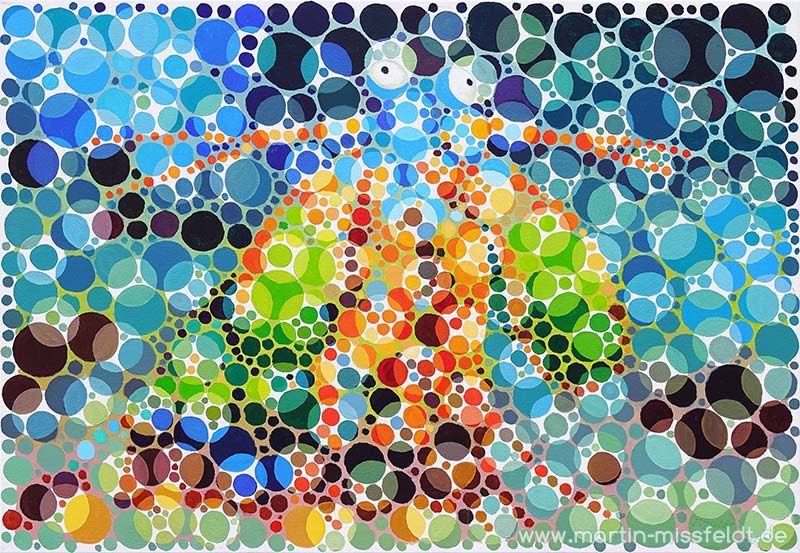This horizontal rectangular image displays a complex and vibrant array of overlapping circles in various colors and sizes, filling the entire frame. The circles are densely packed, creating an intricate pattern that draws the eye across the entire composition. Predominantly, shades of blue and white occupy much of the image, especially around the sides and bottom, transitioning from lighter blues on the left to darker, almost black shades on the right. Centrally, warmer hues like oranges, reds, greens, and some brown and tans dominate, with these colors more prominently displayed in the middle area and extending toward the bottom. Many circles overlap, causing a blending effect where their intersecting colors create new hues, such as light brown when white overlaps brown. Nestled within this colorful arrangement is an abstract representation of a fly, featuring green and lighter green circular patterns on its wings. The image is artistically complex, with a noticeable textual element at the bottom that reads "www.martin-missile-fallot.de".